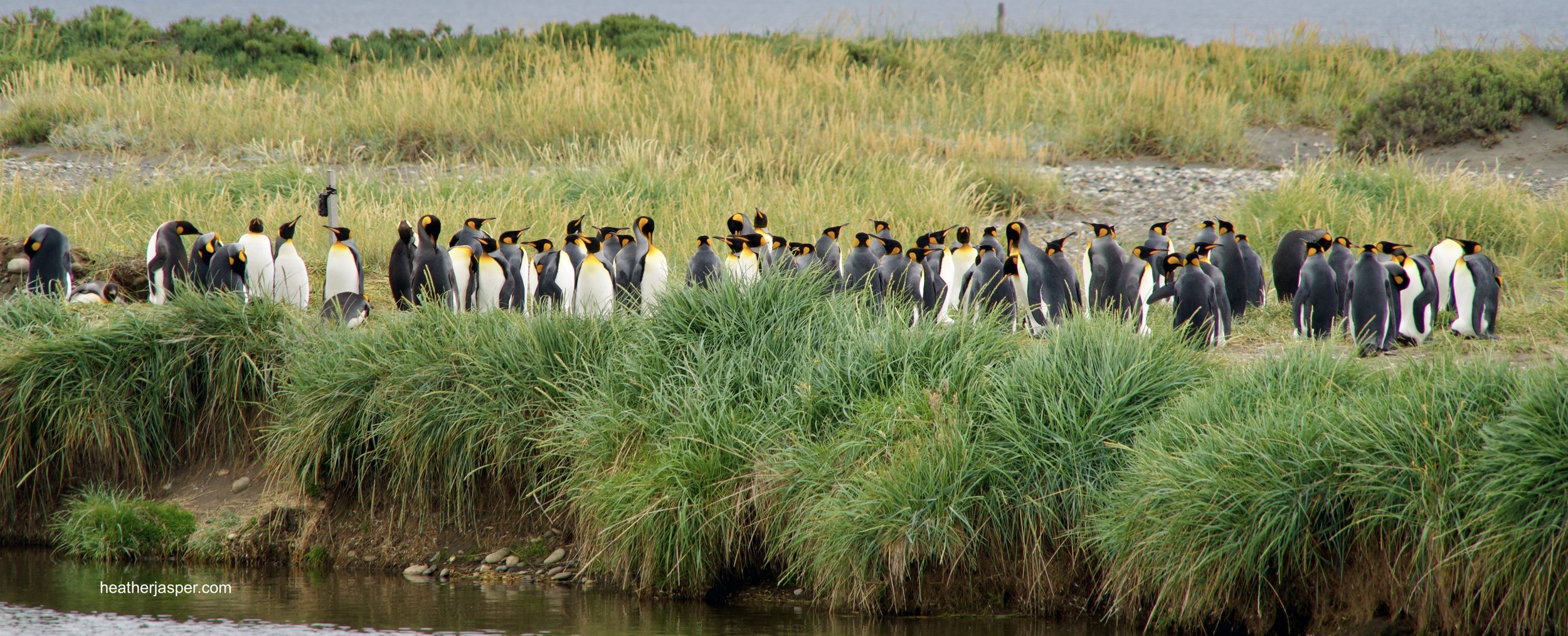The image captures an outdoor scene featuring around 50 large penguins standing in a somewhat orderly line along a riverbank. These penguins, with striking white chests and predominantly black bodies, exhibit a distinctive yellowish-orange patch near their necks and sport pointed yellow beaks. The penguins are depicted both facing towards and away from the camera, revealing either their white breasts or their black backs. The foreground showcases a steep bank leading down to a sliver of visible water, adorned with long, stringy, ornamental-like grass. Behind the penguins, thick clumps of vibrant, bushy grass and smaller green plants extend towards the background, where a larger water body opens up. The very edge of the image at the bottom left corner displays writing that reads "heatherjasper.com," barely legible. The overall setting lacks snow, suggesting a temperate environment.